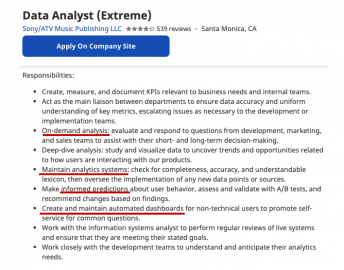**Job Advertisement for Data Analyst Extreme at Sony/ATV Music Publishing LLC**

**Apply on Company Site**

**Responsibilities:**
1. **Key Performance Indicators (KPIs):** Develop, measure, and document KPIs relevant to business needs and internal teams.
2. **Liaison Role:** Act as the main liaison between departments to ensure data accuracy and uniform understanding, critical for the development and implementation teams.
3. **On-Demand Analysis:** Evaluate and respond to questions from development, marketing, and sales teams to assist with both short and long-term decision-making. (Note: "On-Demand Analysis" is highlighted in red in the original document).
4. **Maintain Analytic Systems:** Ensure systems' completeness, accuracy, and clear lexicon, and oversee the introduction of new data points or sources. (Note: This aspect is highlighted in red in the original document).
5. **User Behavior Predictions:** Make informed predictions about user behavior, validate with A/B testing, and recommend changes based on findings. (Note: "A/B Test" is highlighted in red in the original document).
6. **Automated Dashboards:** Create and maintain automated dashboards for non-technical users to enable self-service for common questions. (Note: This responsibility is highlighted in red in the original document).
7. **System Reviews:** Collaborate with information system analysts to perform regular reviews of live systems and ensure they meet stated goals.
8. **Development Teams Support:** Work closely with development teams to understand and anticipate their analytics needs.

**Note:** This is a highly detailed job summary with specific responsibilities underlined for emphasis. Each role is crucial to the efficient functioning of Sony/ATV Music Publishing LLC's data analytics operations. Apply now to join our dynamic team!